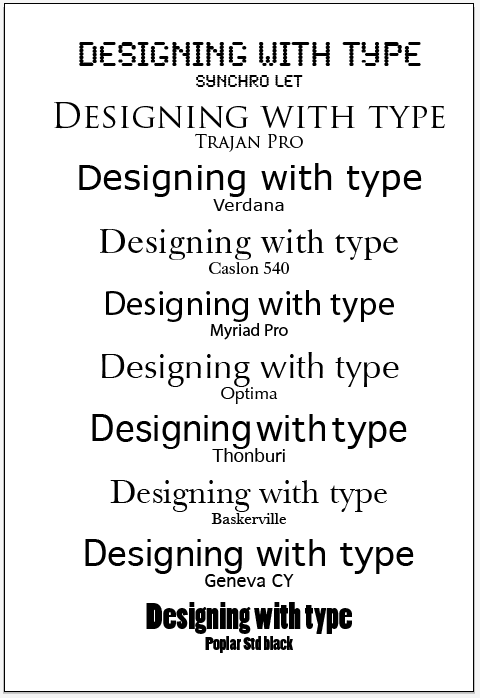The image displays a poster with a white background and a thin black border, showcasing the phrase "Designing with Type" repeated in various fonts. At the very top, the phrase is written in large black letters. Each subsequent line also says "Designing with Type," but in different fonts and with the corresponding font name beneath it. The fonts, in order from top to bottom, are Synchrolet, Trajan Pro, Verdana, Caslon 540, Myriad Pro, Optima, Thonburi, Baskerville, Geneva CY, and Poplar Std Black. Some lines feature all capital letters while others use a mix of uppercase and lowercase. The text is centered horizontally across the page.